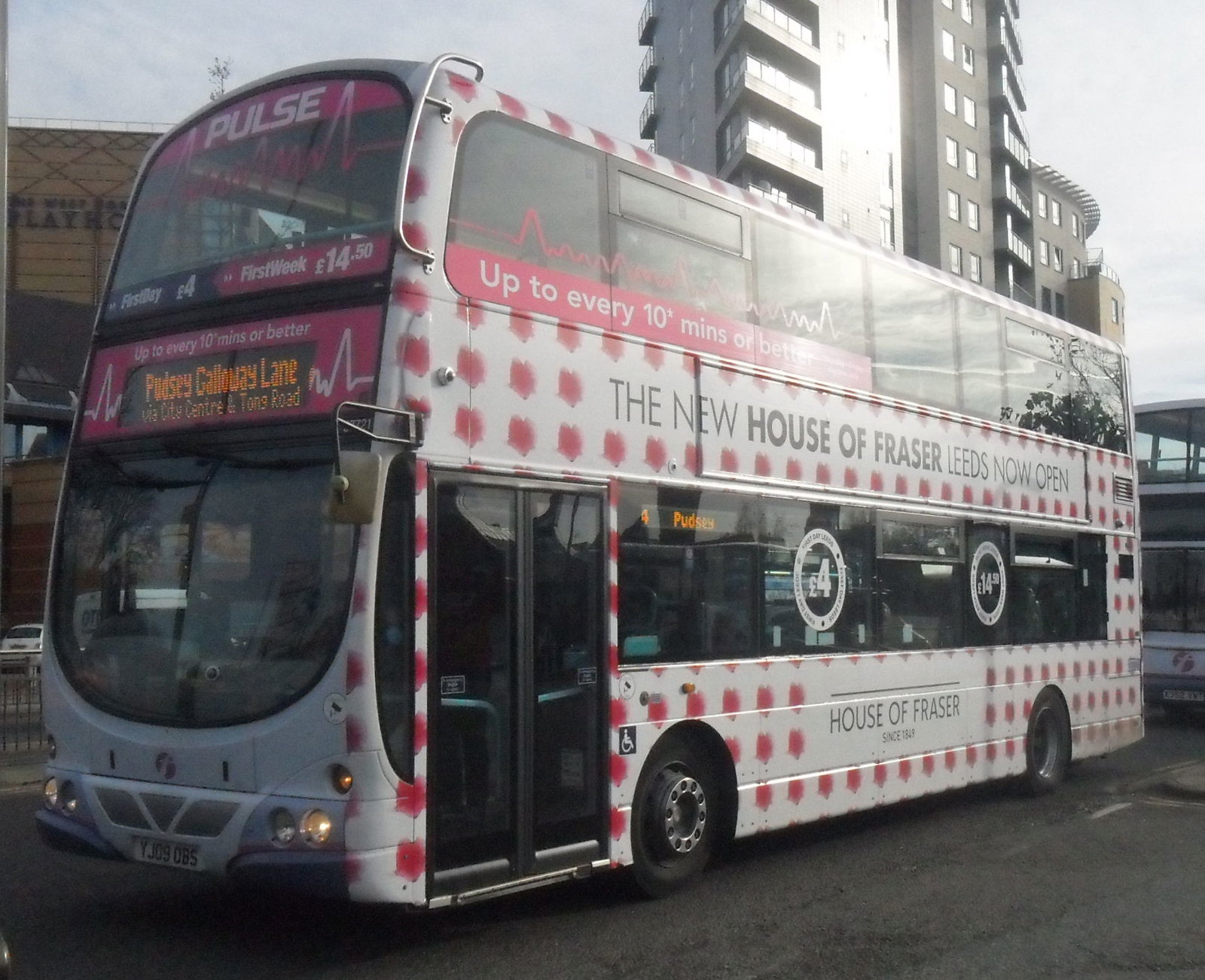The photograph captures a double-decker bus, primarily white with pink accents, parked in a lot under gray skies, possibly in London. The bus prominently features the text "Pulse" in a pink header at the top front, along with a pink line and a white pulse line graphic indicating frequency of service ("up to every 10 minutes or better"). Its route information is displayed with yellow text on a black background, stating "Pudsey Galloway Lane via City Center and Tong Road." The side of the bus features extensive advertising for the "new House of Fraser Leeds now open," with smaller print noting "House of Fraser since 1849" at the bottom. The bus's windows also display promotional content. The reflective windshield and lack of visible driver suggest the bus is empty. The scene includes another double-decker bus behind it, parked on gray tarmac, with a tall building and smaller structures in the background. The bus's lights are on, indicating it's late evening or approaching nighttime.